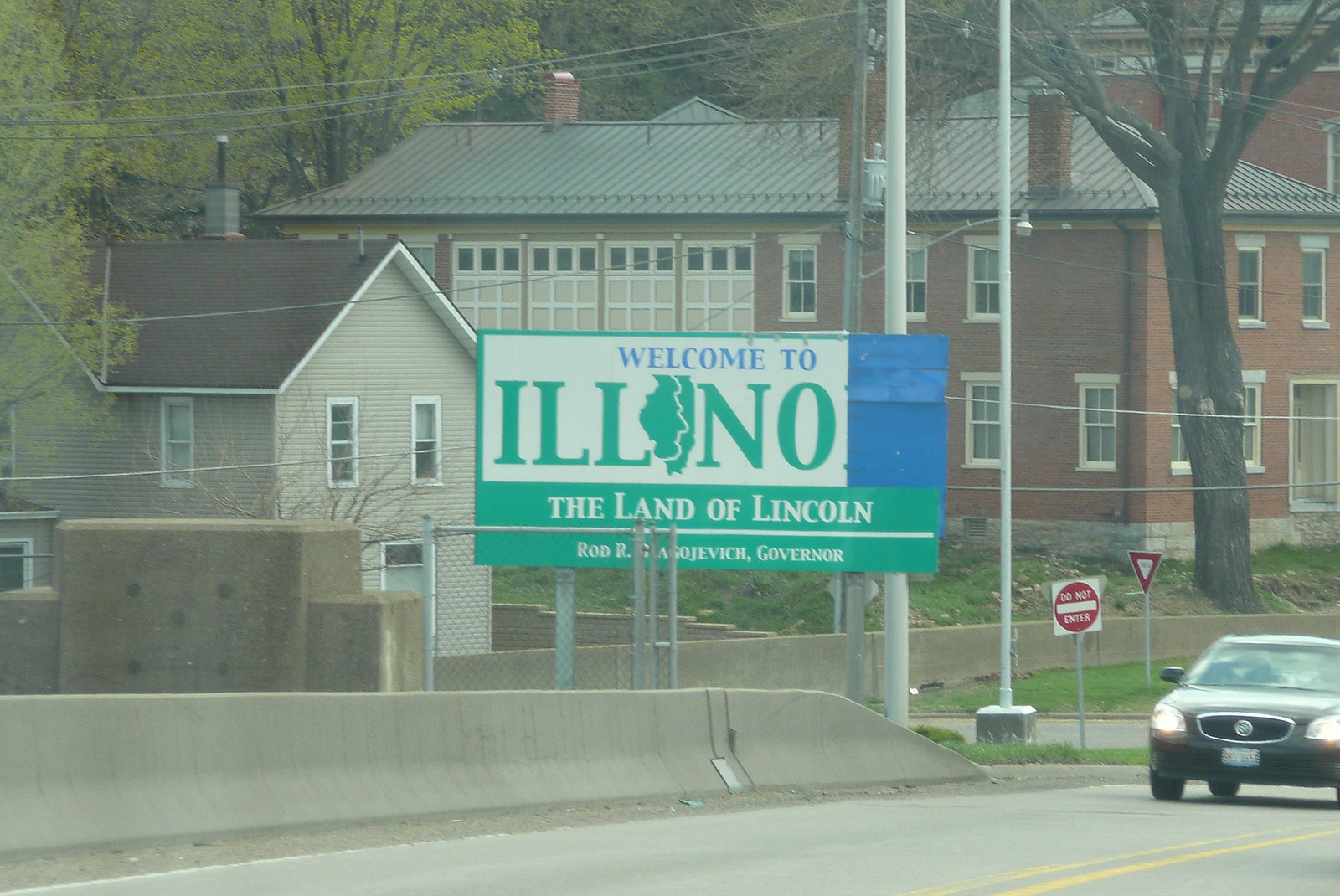This rectangular photograph captures a wide road entering Illinois, prominently featuring a weathered "Welcome to Illinois, The Land of Lincoln" sign at its center. The sign, typically seen at state borders, is partially obscured by blue tape, cutting off the last few letters of "Illinois." The second "I" in "Illinois" is artistically shaped like the state itself. The sign also mentions the governor's name, although it's not fully visible.

A black car with its headlights on approaches on the road. To the right of the road, a large red-brick building, reminiscent of a historic mill or old schoolhouse, stands with numerous windows and a prominent front door. On the left, there is a two-story beige house with brown roofing, possibly an older farm-style structure. Trees dot the background, giving the scene a somewhat residential and small city ambiance. The road between the two buildings indicates that travelers can continue forward and potentially turn left to explore more of the area.